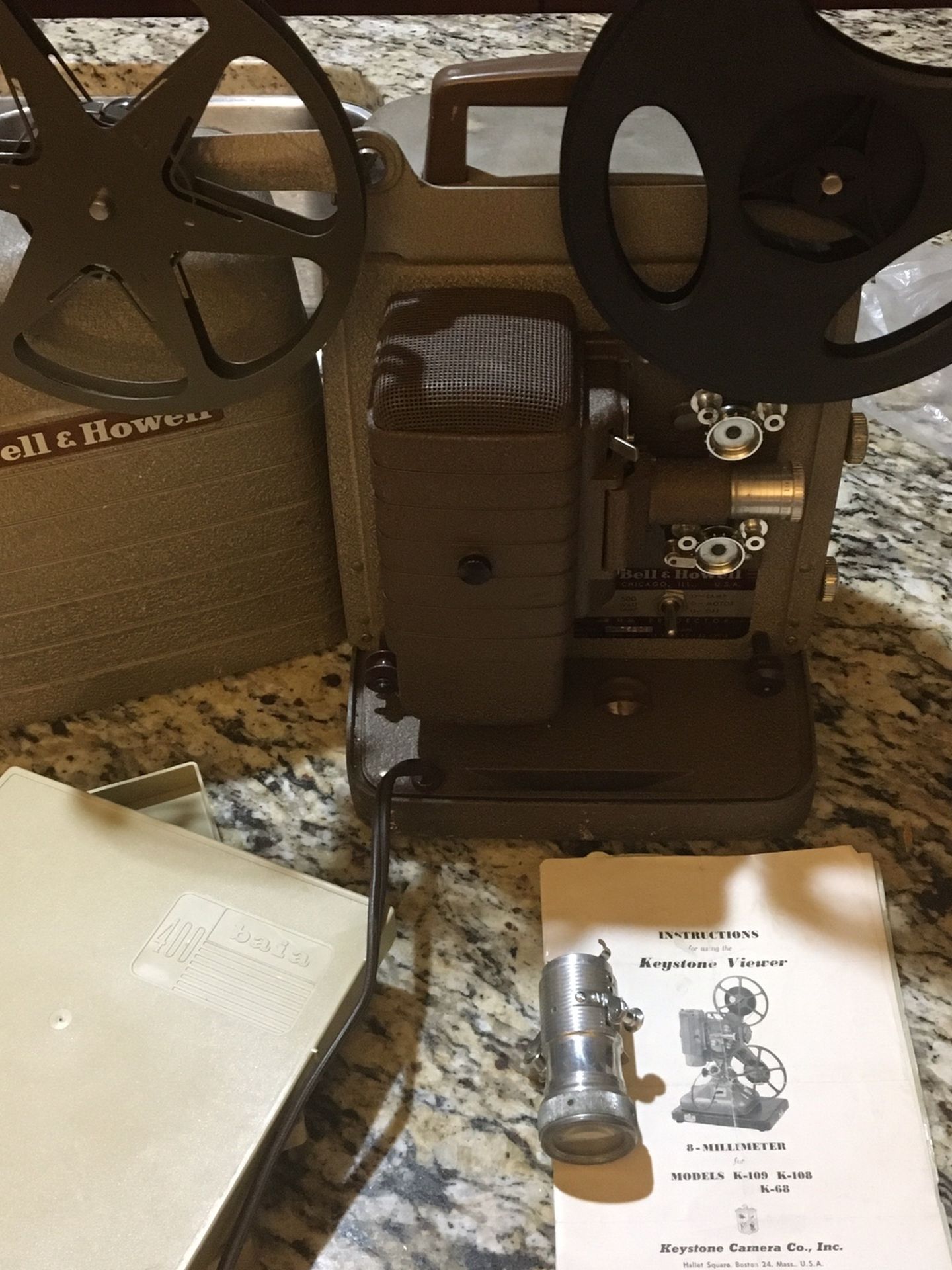The image depicts a vintage Bell and Howell movie projector, prominently displayed on a black and white marble tabletop. The projector features two large reels situated in the top left and top right corners. Between the reels, there are smaller gears and a camera lens embedded in a substantial brown base. Below the left reel, a brown cover is partially visible, displaying the letters "E-L-L" and "Hower," indicating the brand name, "Bell and Howell." The projector is accompanied by a gray and yellow manual positioned at the bottom right of the image, labeled with the word "Instruction" at the top. On top of the manual lies a cylindrical lens attachment or possibly even a long microphone-like piece. Additionally, there is a power cord extending from the base of the projector, trailing out of the frame.